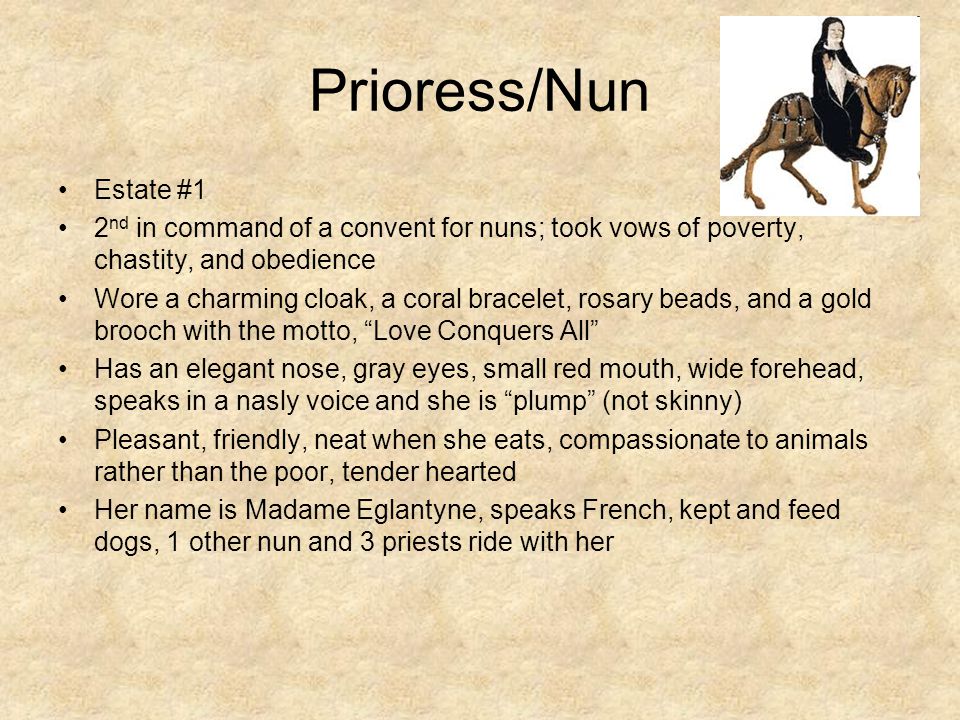The horizontal rectangular image features a decorative beige background resembling aged parchment. In the upper right corner, there is a detailed illustration of a woman riding a brown horse. The woman is identified as a prioress or nun, donned in a black outer garment with a white underlayer. To the left of the image, bold black text reads "Prioress/Nun," indicating a definition is provided. Below the title are six bullet points that paint a vivid picture of the prioress, named Madame Eglantine. 

1. **Estate**: Number one.
2. **Role**: Second in command of a convent for nuns; she took vows of poverty, chastity, and obedience.
3. **Appearance**: She wore a charming cloak, a coral bracelet, rosary beads, and a gold brooch inscribed with the motto "Love conquers all."
4. **Features**: Madame Eglantine is described as having an elegant nose, gray eyes, a small red mouth, and a wide forehead; she speaks in a nasally voice and is plump rather than skinny.
5. **Personality**: She is pleasant and friendly, neat when she eats, and compassionate, particularly towards animals over the poor, displaying a tender heart.
6. **Additional Details**: She speaks French, keeps and feeds dogs, and is often accompanied by one other nun and three priests.